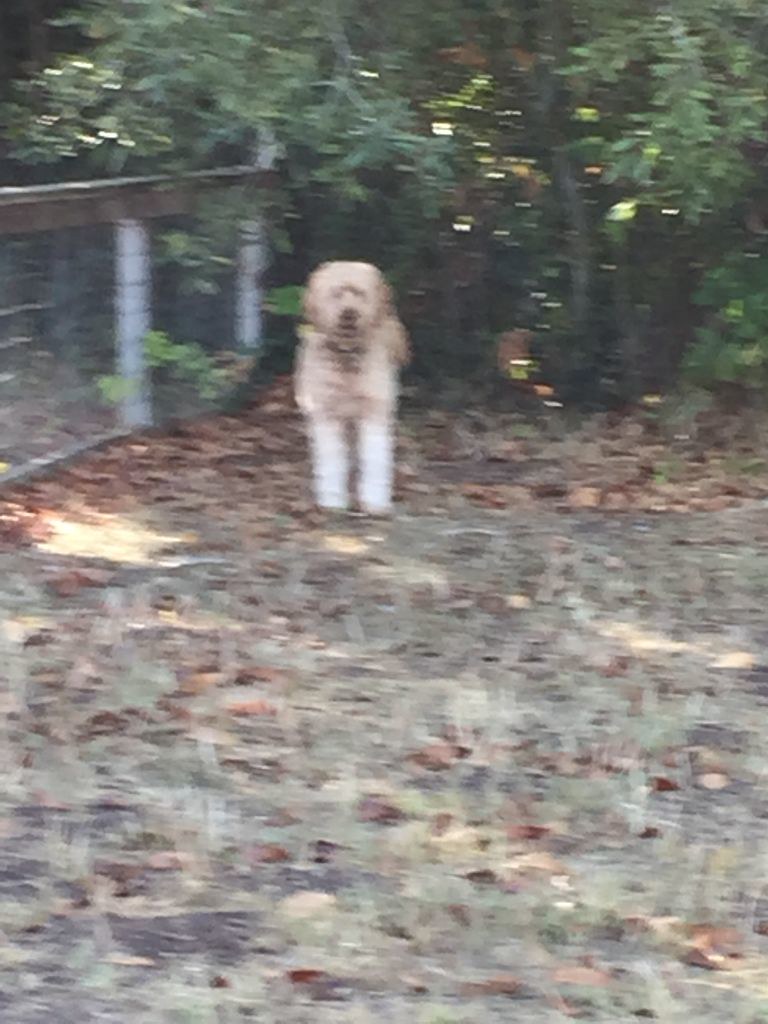A blurry, out-of-focus image captures a tranquil scene where a dog stands in the middle of the frame, seemingly alert and staring forward. The ground is strewn with dry grass and scattered leaves, adding to the rustic atmosphere. To the left, a wooden box is partially enclosed by chicken wire, hinting at a makeshift structure. The background is adorned with a mix of grassy leaves, branches, and trees, with faint sunlight filtering through the foliage, casting a gentle glow on the shaded area. The overall composition, though unclear, evokes a serene and pastoral mood with the dog as the central figure.